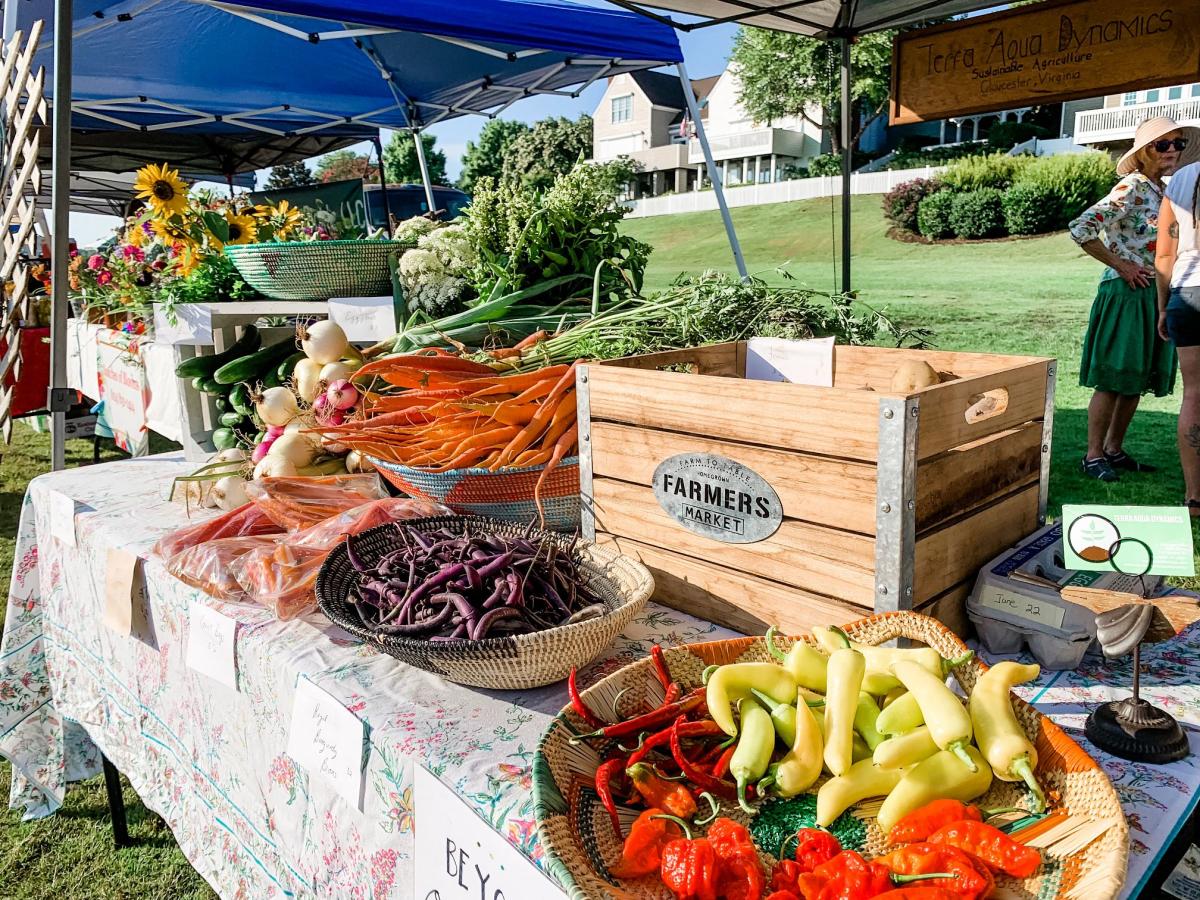The image captures a lively farmer's market set up in a grassy field, framed by several houses in the background. At the forefront, a table neatly covered with a floral tablecloth displays a variety of fresh produce. This table holds several wicker baskets filled with different types of vegetables, including spicy peppers, carrots still bearing their green tops, and cucumbers. A small wooden box on the table, marked "Farmer's Market," stands beside a crate on its side, filled with white and red onions. There's also a basket containing a mix of garlic and zucchini, and a box of eggs can be seen among the colorful array. Adjacent to this vegetable-laden table is another table adorned with a charming green bowl holding sunflowers and tulips, alongside various other vibrant flowers. Both tables are sheltered under tents, providing shade to the displayed goods and creating a pleasant shopping experience. In the background, people, including an elderly woman donning a hat and sunglasses, browse the market, adding life to the scene.